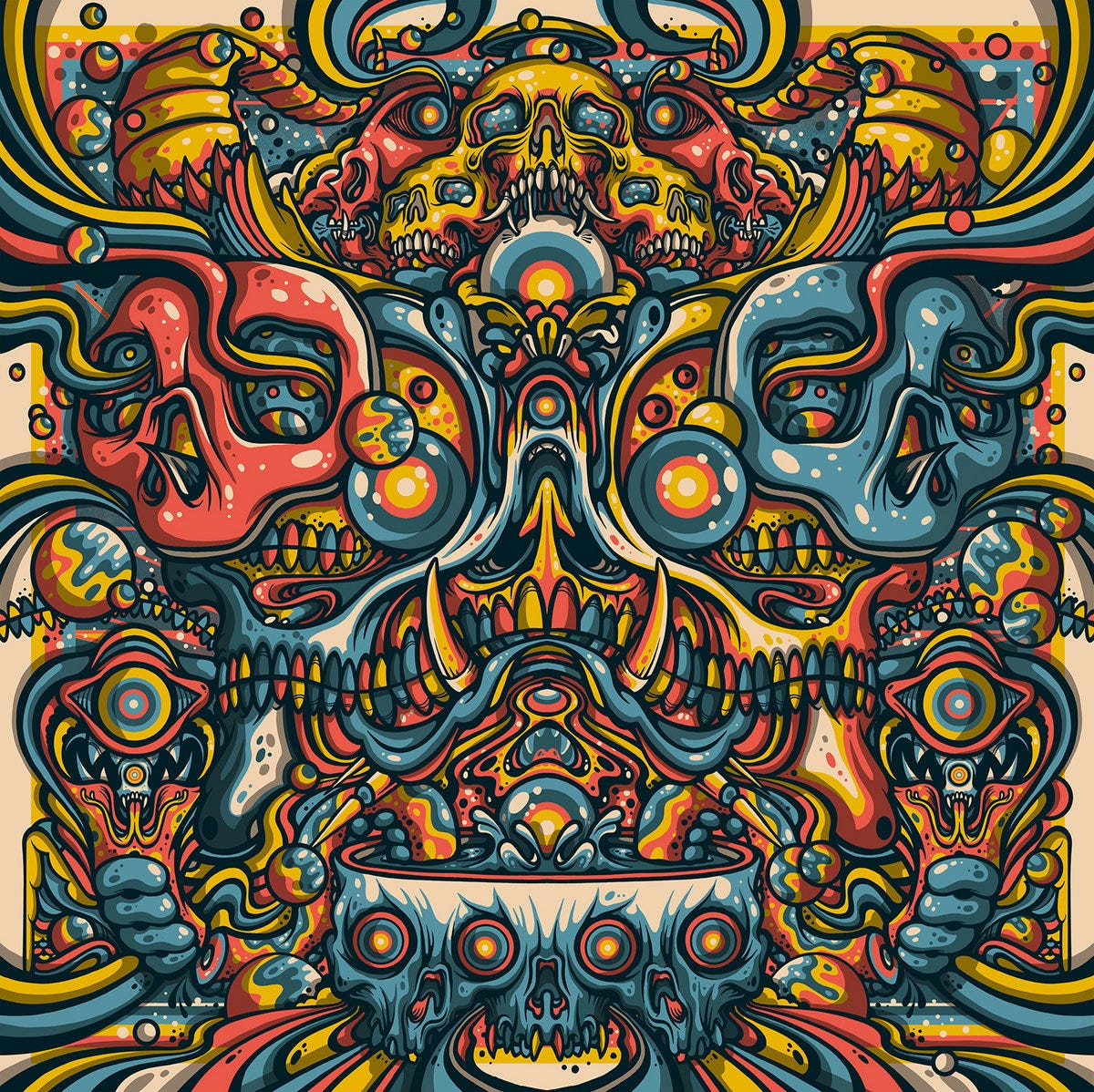The poster is a vivid, multicolored artwork that exudes a fantastical, psychedelic vibe reminiscent of Grateful Dead posters. At its core, it features three prominent skulls: a central gold skull flanked by two others, their eyes glittering with multicolors. Wisps of gold, black, and blue colors swirl across the composition, creating a dynamic sense of movement.

On either side of the central skull arrangement are serpent-like tails, also gold in color. Beneath these are two almost skull-like faces—one in orange on the left and another in blue on the right. Further down, multicolored designs cascade into what resembles a mouth with gold tusks.

This colorful menagerie converges towards a band that looks like a strip of multicolored bullets, flanked by eyes peering down. All these elements seem to flow into a large cauldron at the bottom of the image. This cauldron is decorated with designs of four circles and features a skeletal face with a nose and mouth outlined in similar vivid hues. The artwork is an elaborate explosion of colors—reds, blues, yellows, and oranges—accentuated with stripes, dots, and swirling patterns, all emanating from the central cauldron.